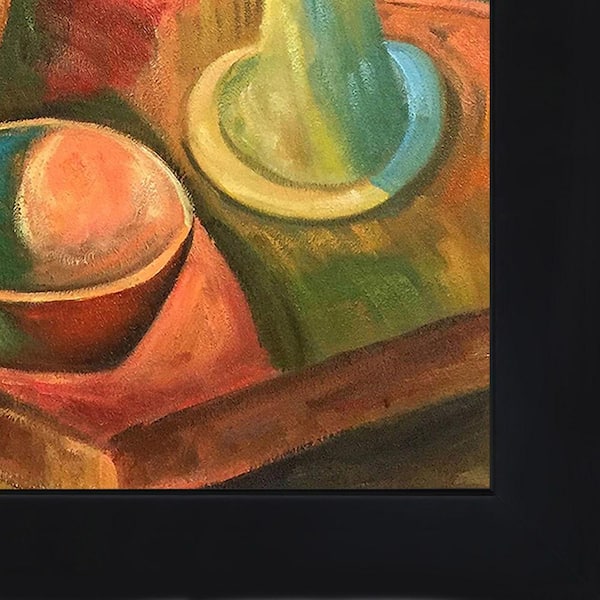The image depicted is the right corner of an abstract still life oil painting, framed by a stark black frame. The painting features a supposed brown table surface, upon which ceramic objects rest. In the left section, there is a bowl with a cream-colored lip, predominantly orange with accents of green. Inside the bowl, a swirl of pale orange, pink, and yellow melds into shades of green and blue. To the right of this bowl stands a cone-like object, with its base on the table; the cone is bisected by color, half yellow and half blue, with the cone's top cropped out of the frame. The background behind these objects consists of deliberate brush strokes forming a straight pattern in vivid hues of orange, green, yellow, and red. The overall scene suggests a still life of ceramic ware, straddling the line between abstract and representational art.